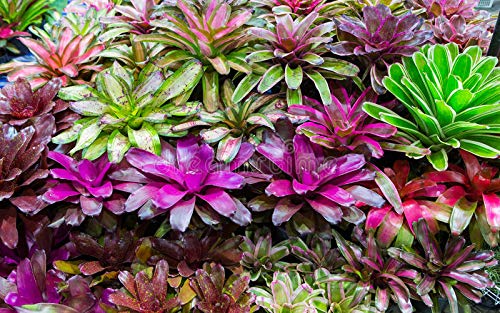In this image, we are viewing a vibrant array of flowers and plants with intricate details and a variety of colors. At the top of the image, there is a stunning mix of vibrant greens, darker purples, and pinks. Moving down to the next row, the buds exhibit green outlines accented with purple specks and fluorescent greens, especially noticeable on the right-hand side. Further down, the blooms display a beautiful gradient of fluorescent pinkish-purple petals with white tips, transitioning to a striking hot pink on the right side. Towards the bottom, the colors become slightly subdued yet still display a harmonious blend of pinks, light reds, and greens, with pink tips accentuating the petals and more pinks concentrated in the bottom right-hand corner. Additionally, the top left section of the image features a unique flower with pink petals and green parts, and there’s a faint inscription in the middle of the picture that reads "Dream Time." The overall composition is rich in color and detail, showcasing a captivating spectrum of greens, pinks, purples, and subtle browns and blues.